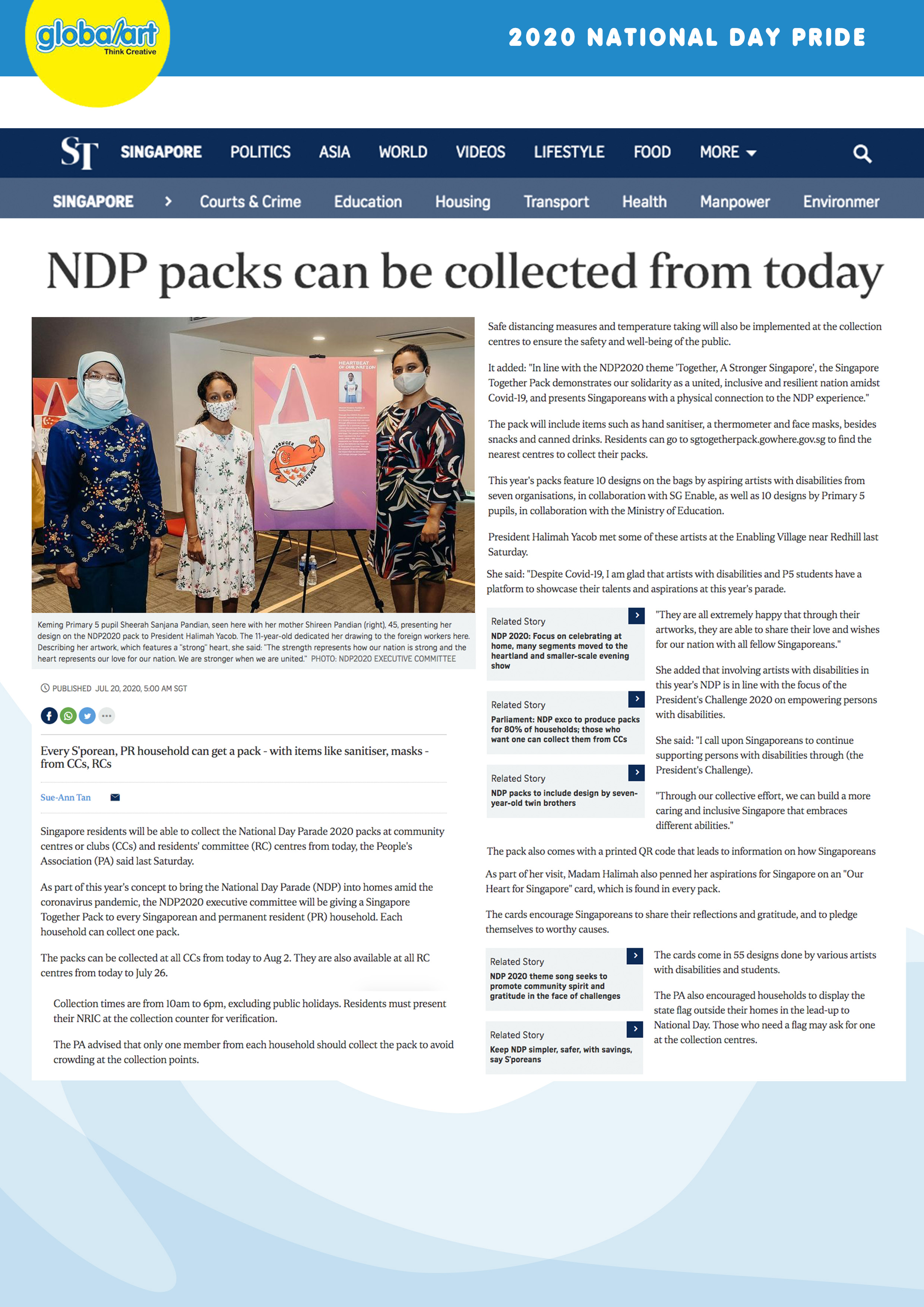A screenshot of a website article is displayed, featuring various interface elements and a detailed scene in the main content section. At the top of the image is a blue horizontal bar. On the left side of this bar is a partially visible yellow circle, about 70% of its full shape, containing decorative text that appears to be a logo, possibly saying "Global Art" in blue and multicolored or blue and white letters. Below this is an unreadable black slogan.

On the right side of the blue bar, in uppercase white letters, reads "2020 NATIONAL DAY OF PRIDE." Below this bar, a white horizontal strip spans across the screen, devoid of any content. Directly underneath it is a black bar containing the primary navigation menu, which begins with "ST." and continues with the following sections in white text: "Singapore" (bold), "Politics," "Asia," "World," "Videos," "Lifestyle," "Food," and "More," with a dropdown menu icon. To the far right is a search icon.

Beneath the primary navigation is a dark gray bar featuring secondary navigation options, starting with a non-bold "Singapore," followed by a greater-than symbol and subsequent sections: "Courts & Crime," "Education," "Housing," "Transport," "Health," "Mango War," and a partially visible "Environment."

The main content area starts with the heading "NDP packs can be collected from today." The article is formatted into two columns. The left column begins with an image of three women indoors, likely in a gallery, all wearing face masks presumably for COVID-19 protection. They appear to be presenting a poster on an easel, depicting a canvas tote bag with artwork and some tiny, unreadable text. The women are described as:

1. The first woman has her head covered and something around her neck.
2. The middle figure seems to be a younger girl in a dress.
3. The third woman also wears a dress and has her hair pulled back into a bun.

They all have dark skin and are standing in front of the tote bag display. Below the image is the caption for the picture, followed by the start of the article text interspersed with social sharing buttons for Twitter and three other platforms that are indistinct.

The article text, in small font, occupies both columns on a white background. The secondary navigation includes a subheading, a dividing line, some blue text, another line, and the main article text. All these sections are set against an abstract, multicolored background featuring shades of blue, white, and light blue.